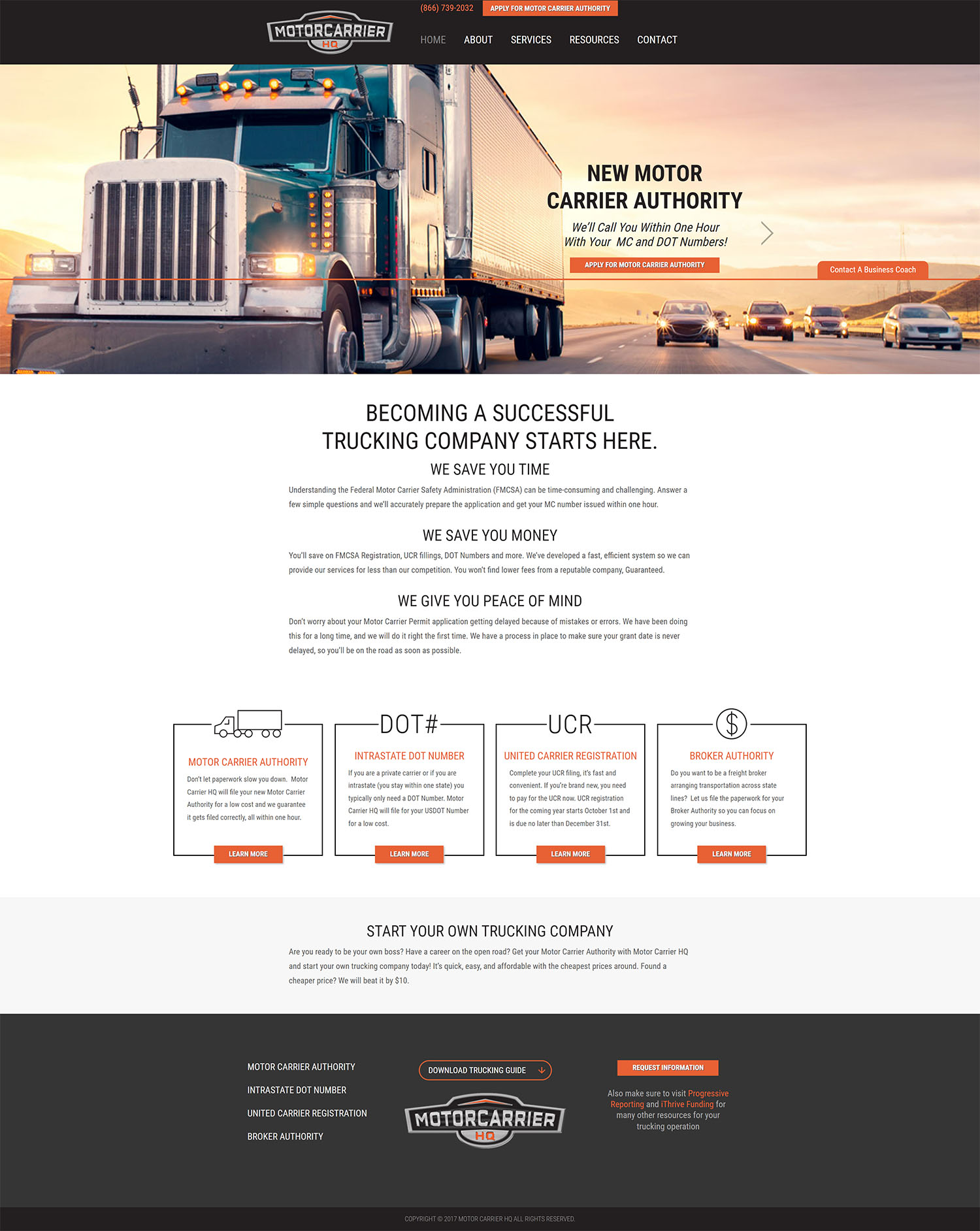The image features a prominently displayed truck traveling on a bustling highway, accompanied by several other vehicles. The context of the image conveys the message: "Becoming a successful trucking company starts here. We save you time, we save you money, we give you peace of mind." Beside the truck, an informational caption states, "New Moto Carrier Authority will call you within one hour with your MC and DOT numbers. Apply for Moto Carrier Authority; contact a business coach." Additionally, the image includes a navigation bar at the top with links to "Home," "About," "Services," "Resources," and "Contacts," while the bottom prominently displays "Moto Carrier HQ."